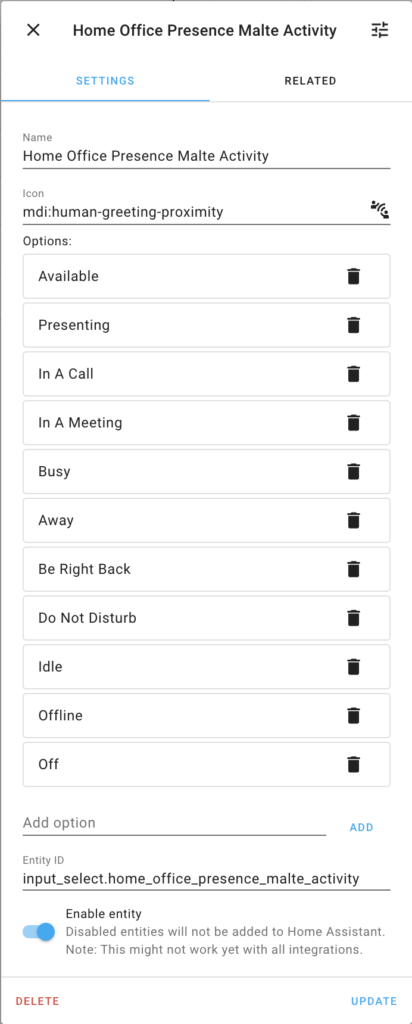A high-resolution screenshot of a smartphone screen displaying a configuration interface for a "Home Office Presence Multi-Activity" setting. At the top, the title "Home Office Presence Multi-Activity" is prominently displayed in black text, flanked by an "X" icon on the left and a triple-line menu icon on the right. Below, two tabs are presented: "Settings," highlighted in blue with an underline, and "Related," in black.

In the "Settings" tab, the label "Name" appears above the text "Home Office Presence Multi-Activity." The following line specifies the "Icon" as "MD: Human Greeting Proximity," accompanied by a small symbol. A horizontal gray line separates this section from the next.

The "Options" section features a series of search bars, each paired with a trash can icon, listing various statuses. These include:
1. Available
2. Presenting
3. In a Call
4. In a Meeting
5. Busy
6. Away
7. Be Right Back
8. Do Not Disturb
9. Idle
10. Offline
11. Off

Beneath these options is the "Add Option" feature, with the word "Add" highlighted in blue, followed by another horizontal line. The field labeled "Entity ID" reads "Input_Select_Home_Office_Presence_Multi_Activity," followed by a black line.

At the bottom of the screen, a light blue switch with a blue circle is labeled "Enable Entity," with a note below stating, "Disabled Entities will not be added to your Home Assistant. Note this might not work with all integrations." The interface also includes two additional options: "Delete" in the lower left and "Update" in the lower right.